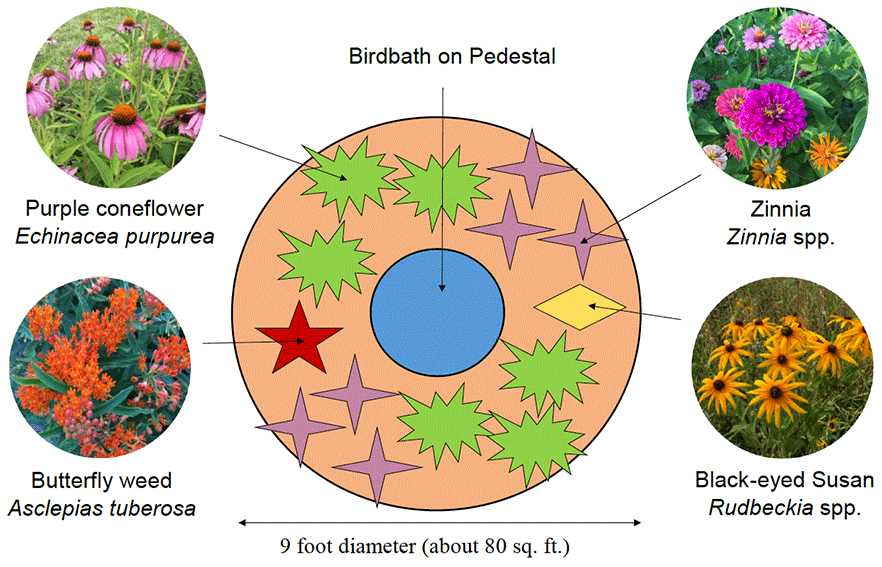The image titled "Bird Path on Pedestal" illustrates a garden layout designed to attract birds, butterflies, and bees. At the center of this cartoonish, top-view map is a round, light tan-orange area. In the middle of this circle lies a blue circle, labeled "Bird Path on Pedestal." Around the central birdbath, different plant zones are marked with various colored shapes: a jagged green shape for Purple Coneflower (Echinacea purpurea) with an actual picture of the flower, a red star for Butterfly Weed (Asclepias tuberosa) accompanied by its photo, a purple cross for Zinnia (Zinnia sp.), and a yellow diamond for Black-Eyed Susan (Rudbeckia sp.), each with corresponding real-life images pointing to the respective planting areas. The garden map specifies a total area of 9 feet in diameter, encompassing roughly 80 square feet.